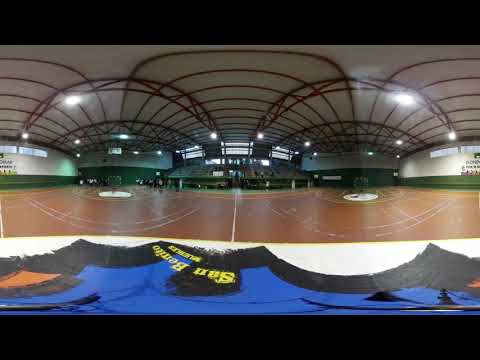This image captures the interior of a large gymnasium. The gym features a chocolate-brown wooden floor with white lines and a white emblem in the center, resembling a basketball court. The floor is divided into two sections, possibly indicating multiple courts. The ceiling is adorned with brown, web-like patterns across a white surface, complemented by numerous bright lights typical of gym lighting. 

In the foreground, on a blue gym floor, lies a white table displaying a blue jersey with black trim and orange accents, featuring partially obscured white lettering that possibly reads "San Bernardino." 

The gym's walls are predominantly white, except for the bottom three to four feet, which are painted green. At the far edges, there are a few bleachers, although they are minimal given the gym's large size. Additionally, structural bracing in red metal supports the roof, giving it a distinctive appearance. 

On the right side of the image, an entryway is visible, along with possible windows or additional writing higher up on the walls. Some distant seating areas, potentially populated with individuals, can be observed, suggesting the presence of spectators. 

Overall, the setting seems to be a multi-purpose sports facility, though no specific sport is immediately identifiable.